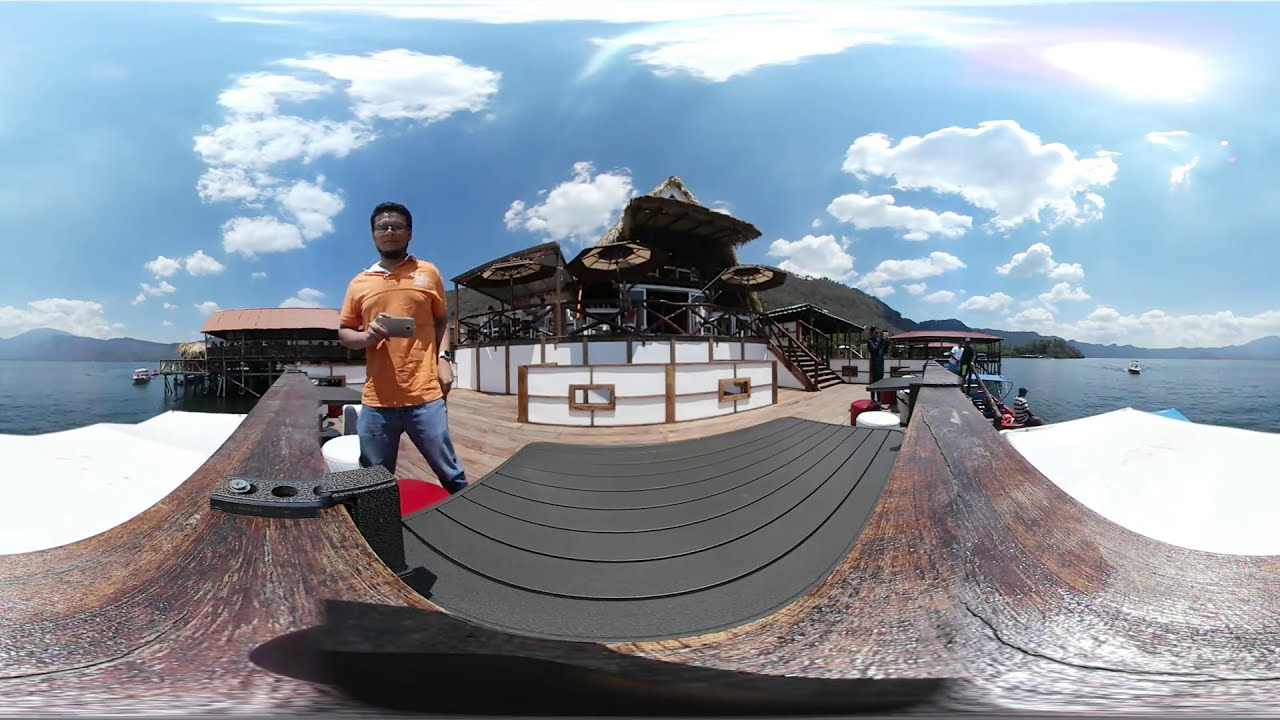In this panoramic color photograph, a young man with dark hair and glasses stands prominently in the foreground, wearing a short-sleeved orange shirt and blue jeans while holding a cell phone in his right hand. The setting appears to be a wooden boardwalk or deck area near a harbor, likely by the sea or ocean, under a sky dotted with scattered cumulus and wispy clouds. The boardwalk features various curves and corrugated surfaces, possibly meant for recreational activities like skateboarding.

Behind the man, there is a two-story building that closely resembles a restaurant or supply port, characterized by its deck lined with several brown and beige umbrellas and tables around the top level. Visible off to the sides, particularly to the right, are boats moored in the harbor and a man fishing nearby. The scene extends towards a body of water framed by distant purple mountains and more visible mountain ranges further back, suggesting a serene but lively coastal environment.

The photograph stitches together three distinct images to create a cohesive panoramic view, with special filters applied for a barrel effect. The landscape captures a mix of natural and man-made elements, portraying a vibrant day with moments of sunlight peeking through the clouds, and a few people scattered around the scene engaging with their surroundings on what appears to be a lively yet peaceful day by the water.